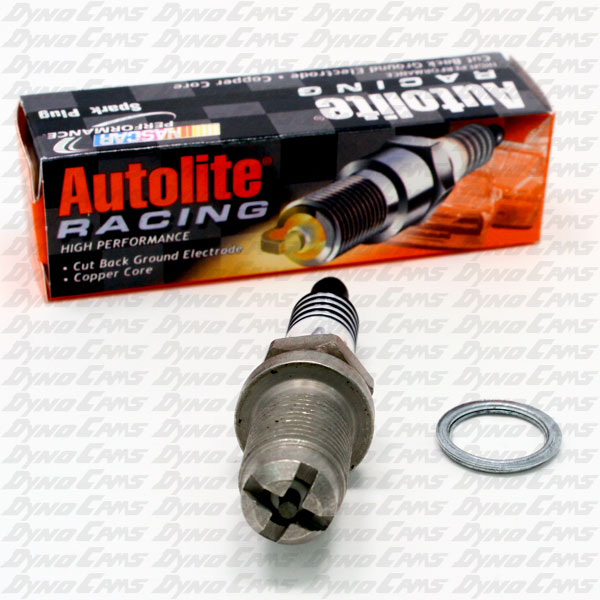A square image features a product against a very light gray background adorned with a repeating, italicized logo reading "DINOCAMS" in light gray all capital letters, arranged in thin rows both horizontally and vertically. The top half of the image showcases a long rectangular cardboard box, predominantly black with accents of red and white, and a black-and-white checkered pattern on the top area. The box is labeled "Autolite Racing" with red text for 'Auto' and blue for 'Light,' and includes additional descriptions such as "High Performance Cut Back Ground Electrode Copper Core." The bottom half of the image displays a round metal tool, presumably a spark plug, accompanied by a small light gray ring to its right. The entire scene is overlaid with the repeated watermark "DINOCAMS," creating a uniform but detailed backdrop.